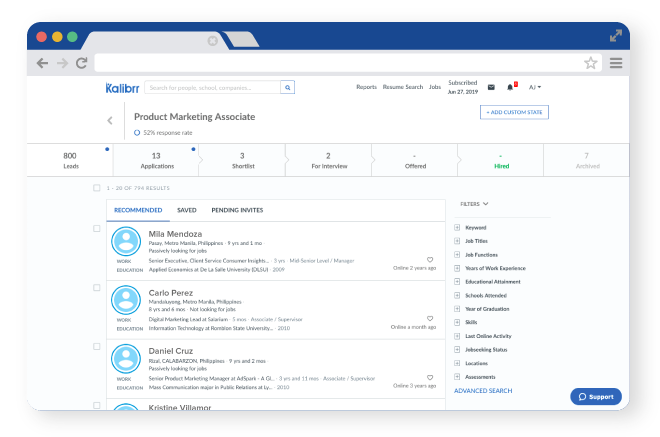This screen capture appears to be from the Caliber (styled as K-A-L-I-B-R-R) website, showcasing a detailed view of various functionalities and interface elements. 

At the top, there's a thin navy strip followed by three colored circles: red, gold, and green. Underneath, there's a gray box with an X on the left, and on the right side, two gray arrows. Moving down, there's a bolded back arrow and a grayed-out forward arrow, followed by a refresh button. Adjacent to these, a white search box is visible, accompanied by a gray star and three lines next to it.

The main body of the screen features a white background atop which "Caliber K-A-L-I-B-R-R" is written in blue. There's another white search box below, with a navy square containing a magnifying glass icon. The interface lists sections labeled "reports," "resume search," and "jobs," along with the subscription date, June 27, 2019. 

To the right, an envelope icon and a bell icon with a red notification dot stand out, alongside a pull-down menu showing "add custom item" in blue. Below this, a summary of a product marketing associate role is displayed, with a 52% metric, 800 leads, 13 applications, 3 shortlisted candidates, and 2 interviews, along with categories like "other" and "mixed."

User information follows, presented on a white background with blue circles displaying white person icons. This section allows users to "recommend" profiles and displays 1 to 20 of what looks like 794 results. There are tabs for "recommend," "saved," and "pending invites."

Beneath the recommendations, names such as Milo Mendoza, Carlo Perez, Daniel Cruz, and Christine Vallemore are listed, each with a gray heart icon indicating how long ago they were online. The interface provides numerous filters for job titles, keywords, and experience levels, wrapped up with an advanced search option in blue at the bottom. Lastly, there's a blue box labeled "invite support."

This comprehensive screen capture illustrates the robust functionality and user interface of the Caliber platform, packed with options for detailed job and candidate management.